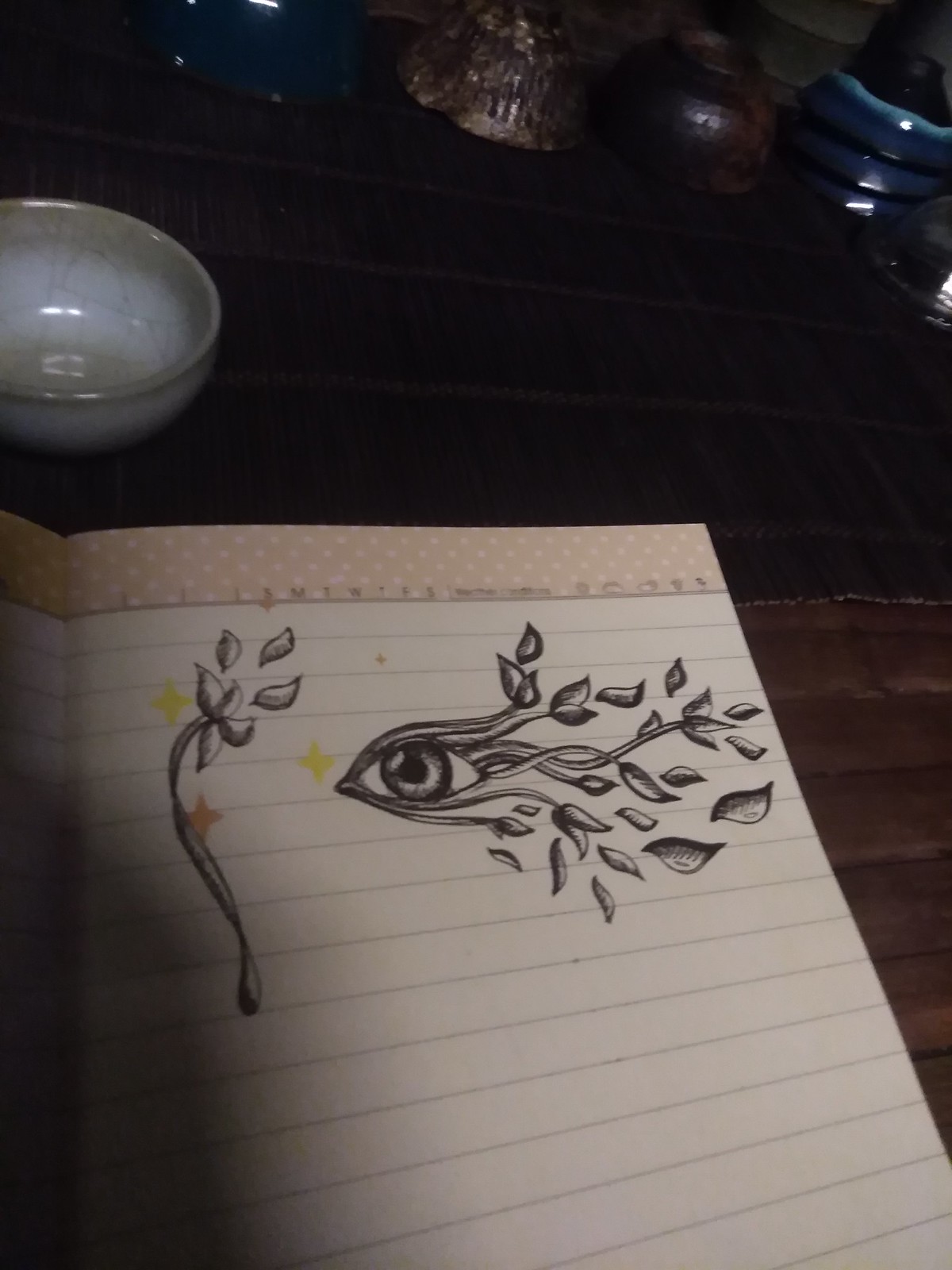In this color photograph, a notebook lies open on a brown table, displaying a detailed pencil drawing on its right-hand page. The notebook paper is white with horizontal gray lines, and the top border is highlighted by a light pink banner adorned with white polka dots. In the upper left corner of the table rests a white bowl, while the upper right features a collection of bowls in varying colors: light blue, dark blue, black, dark brown, beige, and brown. 

The drawing on the notebook's page is an intricate sketch featuring two distinct designs. To the left, there is a depiction of a flower with several petals extending from its stem. To the right, the drawing transitions into an intriguing horizontal eye, surrounded by vine-like stems with leaves growing from and falling off the ends, giving the appearance of an artistic blend between nature and an abstract form.